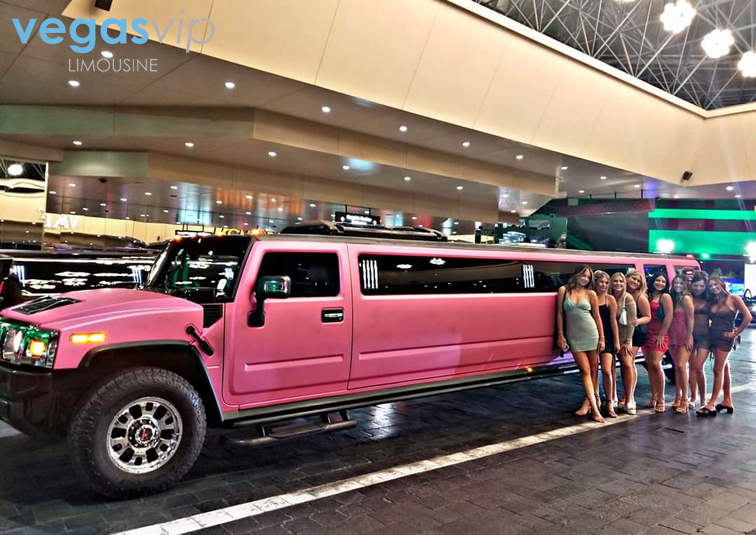The photograph captures a striking pink Hummer limousine parked in a large indoor venue that resembles a car dealership, complete with tall ceilings and dual rafters overhead. The lighting within the space is notable; indented yellow walls feature embedded lights, while additional circular lights are mounted on scaffolding above, casting a white glow over the scene. Adjacent to the limousine, on its right side, is a small crowd of eight women, each donned in club dresses of assorted colors including light greenish blue, black, beige, light red, pink, and brown. Detailed observations reveal one woman wearing a light greenish blue dress with brown hair, another blonde in a black dress, a third carrying a white purse and clad in beige, followed by another blonde also in a black dress, and several others with varying hair colors and dresses in shades of light red, pink, and brown. The limousine has its headlights on, adding to the overall vibrant atmosphere. Additionally, the words "Vegas VIP Limousine" are visible in the top left corner of the image, alluding to a possible advertisement for luxury transportation services. The ground features brick pavers with painted traffic lines, suggesting designated areas for vehicle drop-offs and pick-ups, further indicating that the setting could be associated with a high-end casino or dealership environment.